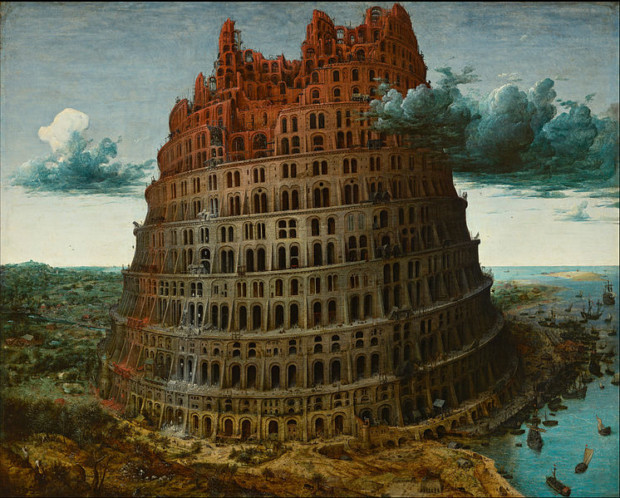This is a detailed painting of a large, fantasy tower that evokes the Tower of Babel, with a structure that resembles the Coliseum. The tower has seven distinct levels and an eighth level that appears under construction. The circular design tapers slightly as it ascends, each level smaller than the one below. At the top, the stone changes from gray at the base to a reddish hue at the unfinished upper levels, characterized by broken arches and incomplete sections.

The tower is positioned on a tan surface, bordered by a body of water on the right side. In the water, small boats—sailboats and cargo boats—are seen faded, adding to the historical and epic atmosphere. The left side of the scene includes a landmass with trees, providing a natural contrast to the imposing man-made structure. The sky around the tower is semi-cloudy with clouds hovering just below the top levels, adding a mystical element to the composition and emphasizing the tower's enormous scale.